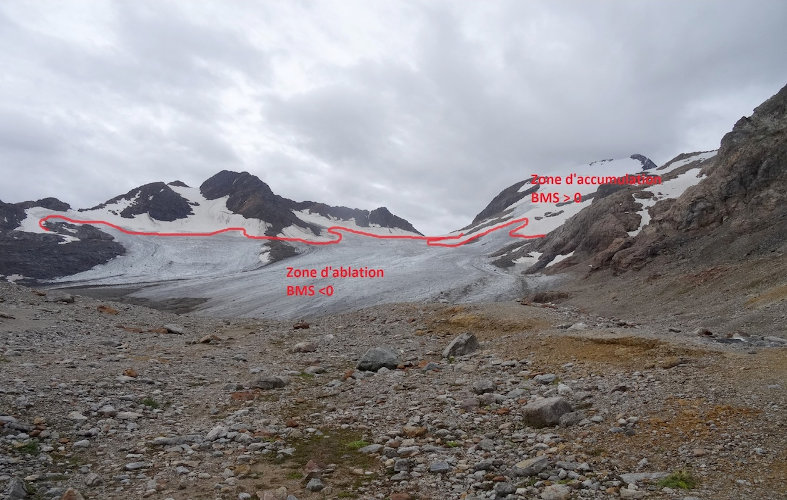In this daytime photograph, we are presented with a striking close-up view of a mountainous landscape. The foreground is dominated by a gravelly area scattered with rocks and patches of moss. Beyond this, we see a ridge leading up to partially snow-covered mountains. A prominent and somewhat meandering red line is drawn about halfway up these landforms, marking a contrast between two zones. This line, not perfectly straight, flows in ripples across the terrain, sometimes rising and falling with the contours of the mountains. 

The line serves as a boundary, with distinct red lettering labeling two areas. To the left and lower portion of the line, it reads "Zone de-ablation, BMS < 0," indicating the zone of ice melting. Higher up and to the right, on the snowier peaks, it is marked "Zone de-accumulation, BMS > 0," designating the area where snow accumulates. The sky above is overcast, a blend of white and blue tones with dense cloud cover, adding a dramatic backdrop to the rugged, icy expanse below.